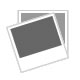The image depicts a complex device featuring a metallic pole or rod that emerges from the top left at an angle. The rod curves downward, then horizontally along a white surface. Behind this silver pole, part of a white sheet or cover is visible. Attached to the pole is a white component with wires and a small red bubble indicator. To the side of the main pole, a black object with a red dot connected to the device is noted. The bottom of this black object features a central piece.

In the top right corner of the image, there is a red bubble labeled "2" with text reading "Nitrile rubber foam, sturdy and durable." The bottom left corner shows a red box containing a white device, with an associated red circle labeled "1" and text stating, "Silver palladium alloy, accurate readings, high durability." The background is partially obscured by a blurred metallic structure.